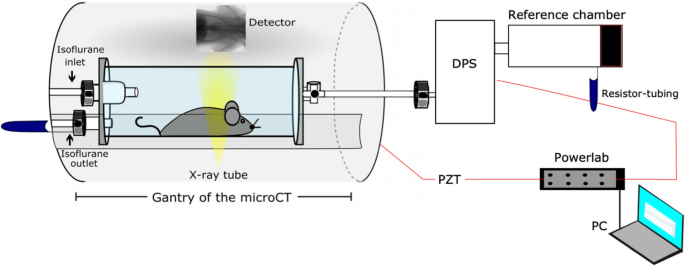The detailed illustration is a scientific diagram of a micro-CT gantry setup. On the left side, a barrel-shaped X-ray tube lies on its side, labeled "gantry of the micro-CT," with the top part marked as "detector." Inside the barrel, there’s a tube containing a mouse. The left side of the mouse is connected to tubes labeled "isoflurane inlet" and "isoflurane outlet," suggesting an anesthesia setup. To the right, another tube connects the barrel to a flat text box labeled "DPS." Adjacent to the DPS is a sideways rectangle labeled "reference chamber," which is half black and half white. Beneath this setup is a blue component labeled "resistor tubing." A red line connects the DPS, resistor tubing, and the barrel to a labeled "power lab," which in turn is connected to a laptop PC. Additionally, the setup includes components labeled as PZT. The drawing features accents in colors like gray, lilac, and turquoise, with yellow light shining on the mouse, representing a detailed and intricate scientific experimental setup.